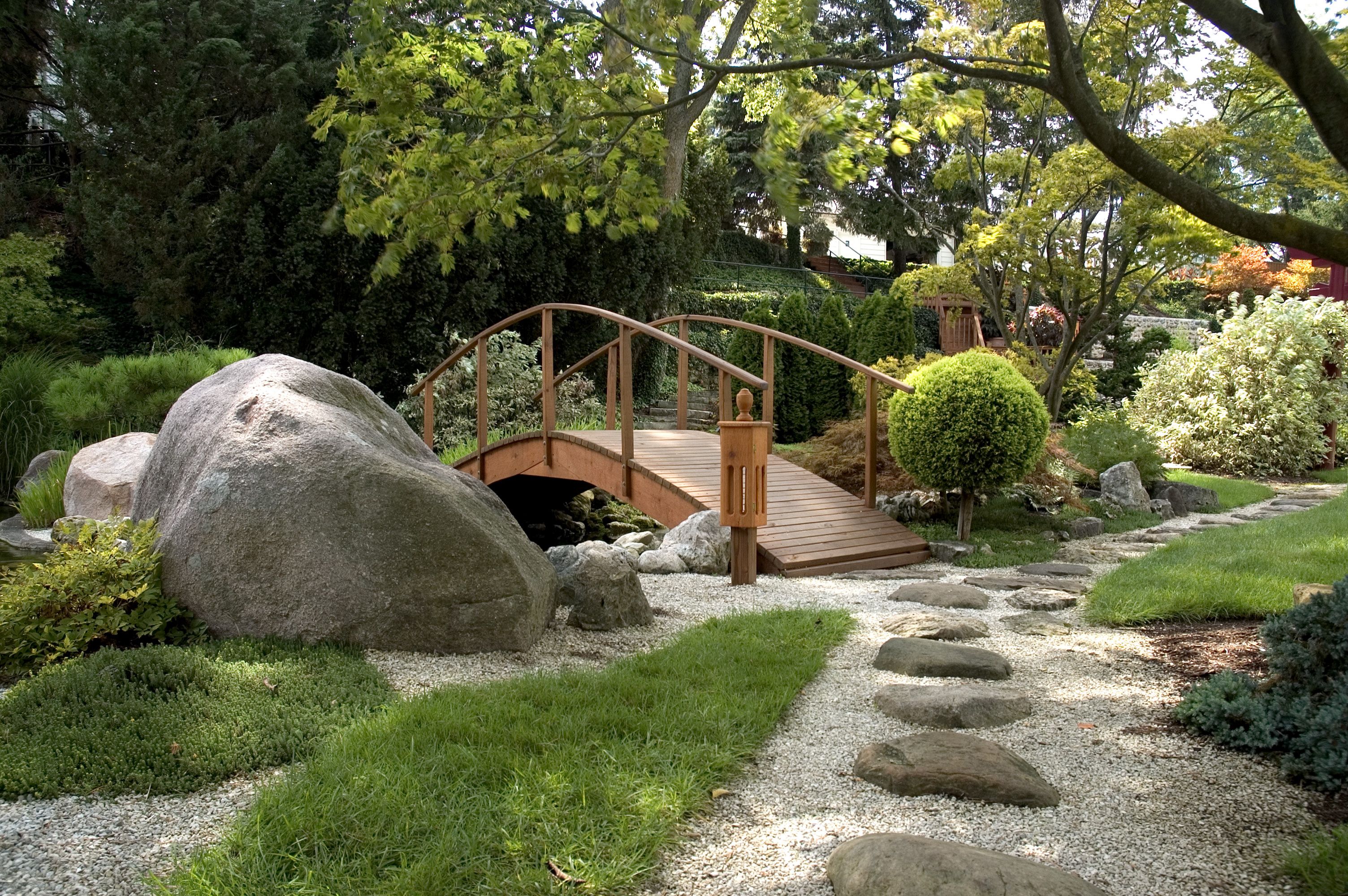In the photograph, we see an intricately designed Japanese-style garden that exudes a serene, Zen ambiance. The garden features a beautifully arched wooden footbridge located centrally, painted a rich brown and equipped with arm handles on either side. The bridge traverses a small body of water, likely a pond or stream, adding to the tranquil atmosphere. The garden path meanders through the lush greenery, formed by a combination of light grey gravel and asymmetrically placed dark grey stepping stones. This deliberate arrangement of stones enhances the natural yet meticulously curated aesthetic of the space.

On the left side of the garden, a large grey rock anchors the scene. Nearby, various plants and bushes have been artistically sculpted, with one notable bonsai-like plant featuring a rounded top resembling a green ball atop a slender stem. The grass in the garden is rich and green, though less uniformly mowed, contributing to its organic appeal. Alongside the path and bridging the spaces between the greenery, a diverse array of bushes, trees, and other plants extend into the distance. These include meticulously manicured trees that blend a sense of naturalness with careful cultivation.

In the background, the dense foliage gives way to glimpses of blue sky, framed by the towering trees and bushes that define the garden's perimeter. The layout and elements within the garden – from the stepping stones and gravel path to the diverse plant life and central bridge – collectively deliver an authentic Zen garden experience, characterized by its peaceful and contemplative design.